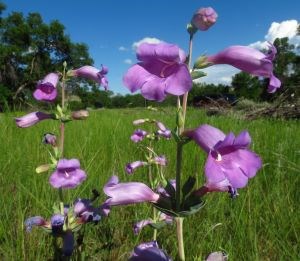This detailed color photograph captures a lively meadow scene, showcasing a trio of tall, green-stemmed plants adorned with delicate, purple trumpet-shaped flowers, some with white centers. The flowers in the immediate foreground vary in their blooming stages - some are fully open, displaying their petals proudly, while others remain buds. Notably, the plant closest to the viewer has five flowers, including one at the top that's still closed, while the plant on the left further back boasts more flowers that are less open. The meadow itself brims with long, lush green grass, lending a slightly wild appearance. Encircling the meadow, a dense array of trees with dark green leaves frames the scene, and a pile of logs and sticks can be spotted to the right in the distance. Above, a richly blue sky almost completely free of clouds provides a serene backdrop, with a few white, puffy clouds dotting the horizon and enhancing the overall tranquility of the landscape.